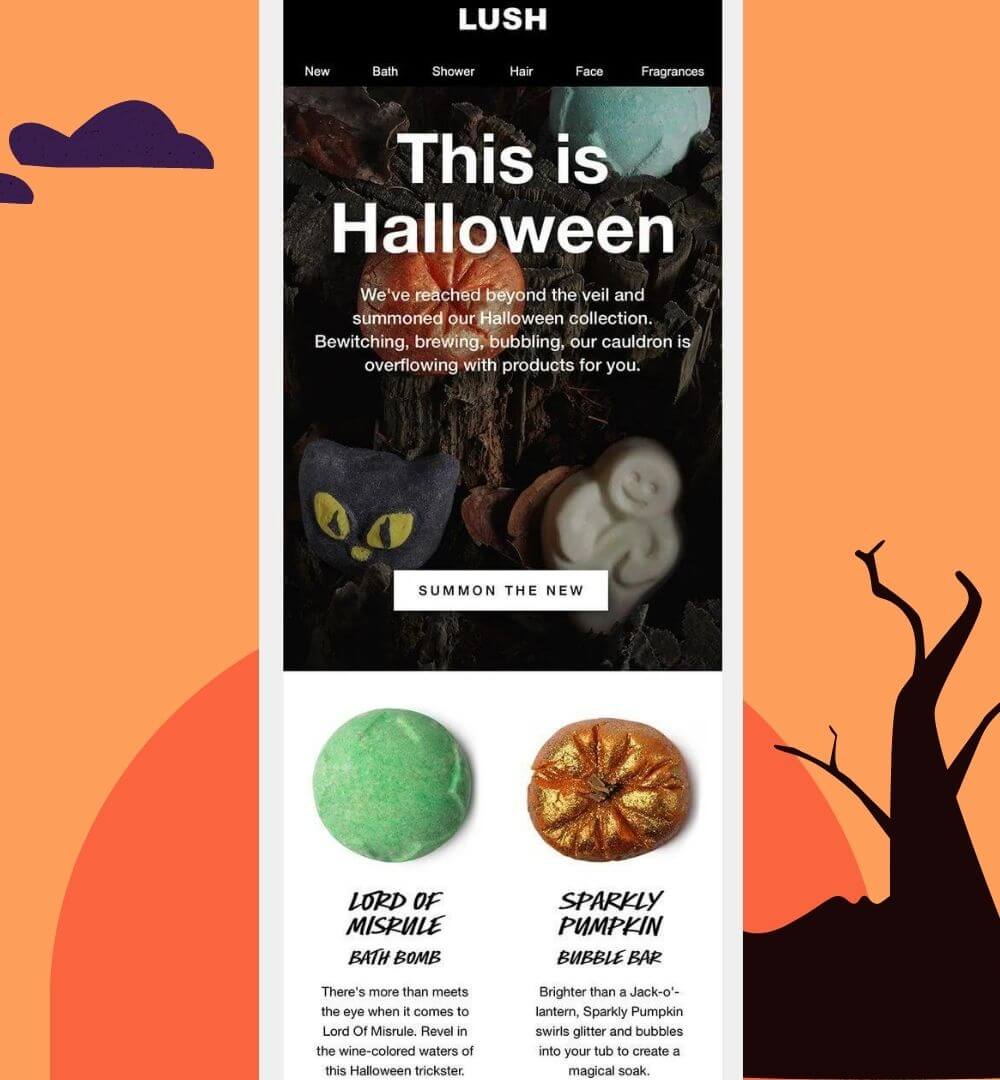Screenshot from the Lush Brand Webpage Showcasing Their Halloween Collection

In this captivating screenshot from Lush's official webpage, the center prominently features an enticing announcement: "This is Halloween, we've reached beyond the veil and summoned our Halloween collection. Bewitching, brewing, bubbling, our cauldron is overflowing with products for you." Beneath this mystical proclamation is a call-to-action inviting users to "summon the new."

To the left, the spotlight shifts to the "Lord of Misrule" bath bomb with an intriguing caption: "There's more than meets the eye when it comes to Lord of Misrule. Revel in the wine-colored waters of this Halloween trickster." Adjacent to this description is the "Sparkly Pumpkin" bubble bar, celebrated for its magical transformation: "Brighter than a jack-o-lantern, Sparkly Pumpkin swirls, glitters, and bubbles into your tub to create a magical soak."

The background of the screenshot adds to the Halloween ambiance with an animated illustration featuring a radiant sun, an orange backdrop, and a couple of silhouetted trees. The entire visual is elegantly enclosed within a rectangular frame, enhancing the festive allure.

Thank you for watching.